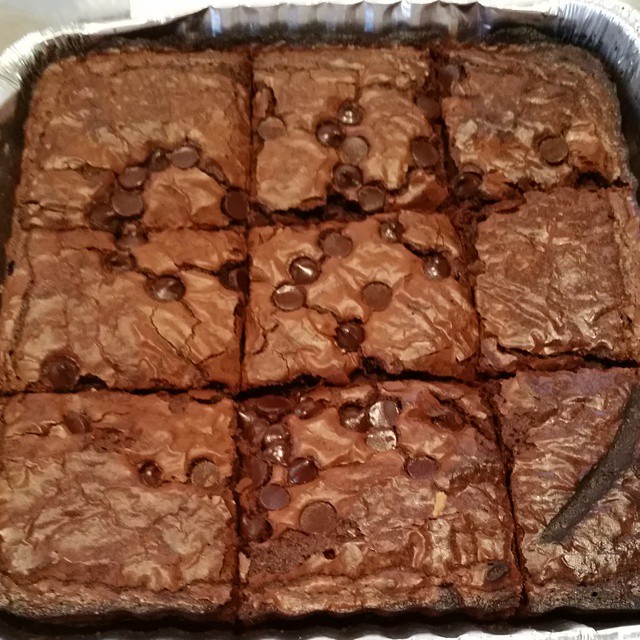This is a close-up color photo of a tray of chocolate chip brownies baked in a disposable aluminum baking pan, likely 8x8 inches in size. The pan is wrinkly around the edges, typical of thick tinfoil one-time-use trays. The brownies have been cut into nine pieces, arranged in three rows of three. Each brownie has an uneven distribution of chocolate chips pressed into the crinkly tops. The edges of the brownies appear crispy and possibly over-baked, with a darker, slightly burnt appearance. Notably, the brownie in the bottom right corner has a distinct burnt gash running diagonally. In the background, the upper left corner of the image shows a blank white wall or some empty space, keeping the focus firmly on the tray of brownies.